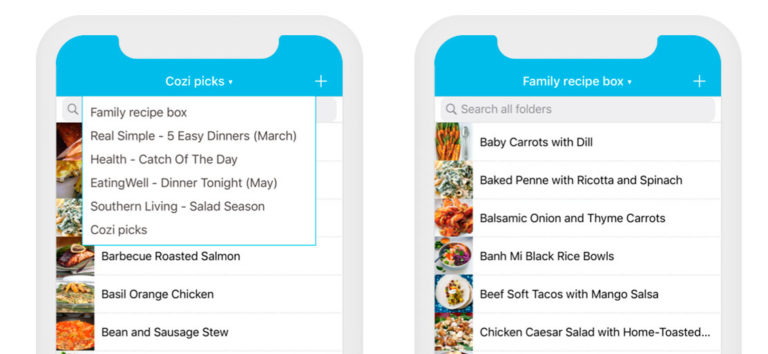The image displays two smartphones, each with a gray border. The smartphone on the left has a blue header displaying "CozyPix" along with a drop-down menu that lists various food categories: "Family Recipe Box," "5 Easy Dinners in March," "Help-Catcher Today," "Eating Well - Dinner Tonight," and "Southern Living Salad Season (May)." Below this, the screen highlights recipe titles including "BBQ Roasted Salmon," "Basil Orange Chicken," and "Bean and Sausage Stew."

On the right smartphone, the blue header reads "Family Recipe Box," accompanied by a search bar labeled "Search All Folders." Underneath, several recipes are listed with accompanying images of each dish. The dishes shown include "Baby Carrots with Dill," "Baked Penne with Ricotta and Spinach," "Balsamic Onion and Thyme Carrots," "Banh Mi Black Rice Bowls," "Beef Soft Tacos with Mango Salsa," and "Chicken Caesar Salad with Home Toasted Croutons."

The detailed visual display on both smartphones highlights a variety of appetizing recipes, ideal for meal planning and diverse culinary preferences.